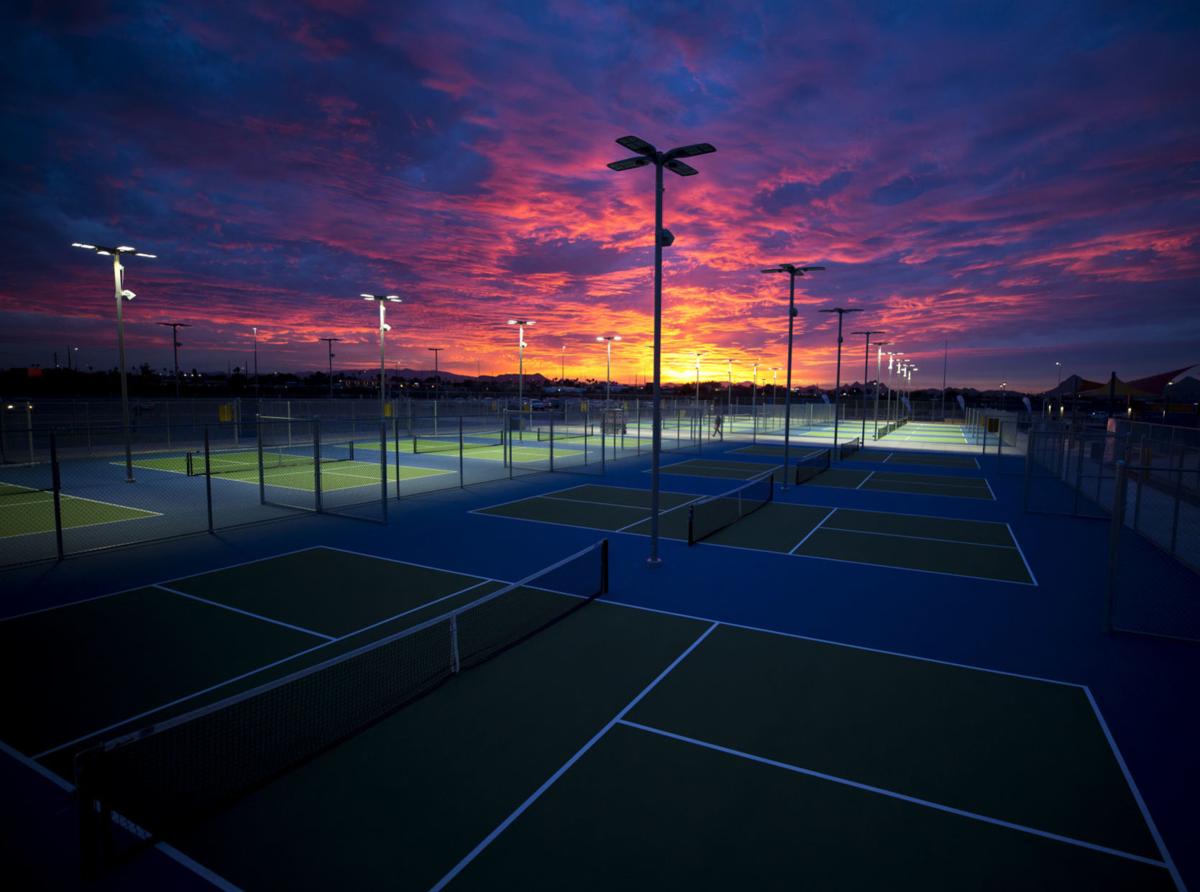The image captures a serene nighttime scene of an expansive tennis court complex as viewed from an elevated position. The vast gated area features at least a dozen side-by-side tennis courts, stretching into the distance, with some estimates suggesting there might be as many as twenty to thirty courts. Each court is bordered by a fence and illuminated by lampposts, though the lighting is uneven—some courts are brightly lit while others remain dark. The courts themselves are characterized by blue perimeters and green playing surfaces, marked off with white lines. In the foreground, a single person can be faintly observed walking between the courts, emphasizing the otherwise complete emptiness of the scene.

Dominating the backdrop is a magnificent sunset. The sky is a kaleidoscope of vibrant colors—pink, yellow, orange, and blue—indicative of the sun just having set. The darkening sky is interspersed with clouds ranging from purplish hues to dark blue, adding to the tranquil yet slightly melancholic atmosphere. In the distance, a row of buildings barely visible, with some lights on, contributes a subtle, urban context to the overall serene image. For more information visit www.FEMA.gov.